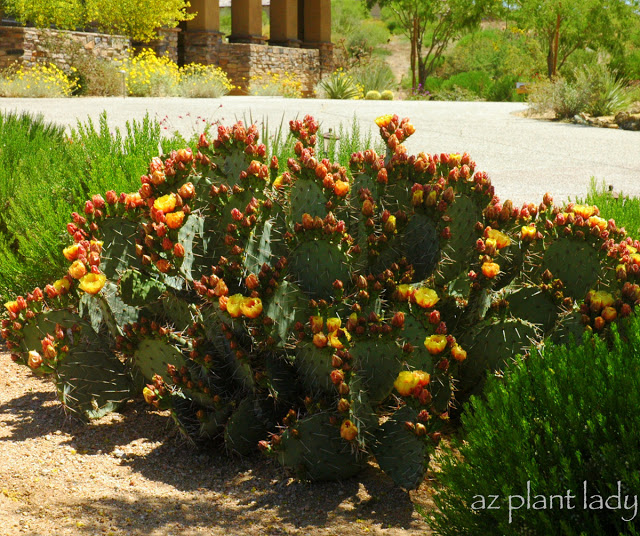The photograph captures an outdoor scene featuring a unique green cactus-like bush adorned with vibrant red and yellow flowers around its edges, resembling yellow tulips. The cactus bush, which is covered in thorns, is flanked by more classic dark green plants on either side. In the foreground, the sandy, yellowish ground contrasts with the lush greenery. The background reveals a large, stone-colored walkway or road leading to a brick building composed of brown, white, and gray bricks. This building features four prominent columns at the front and is surrounded by hills, trees, and various bushes, giving a natural, serene ambiance to the scene.